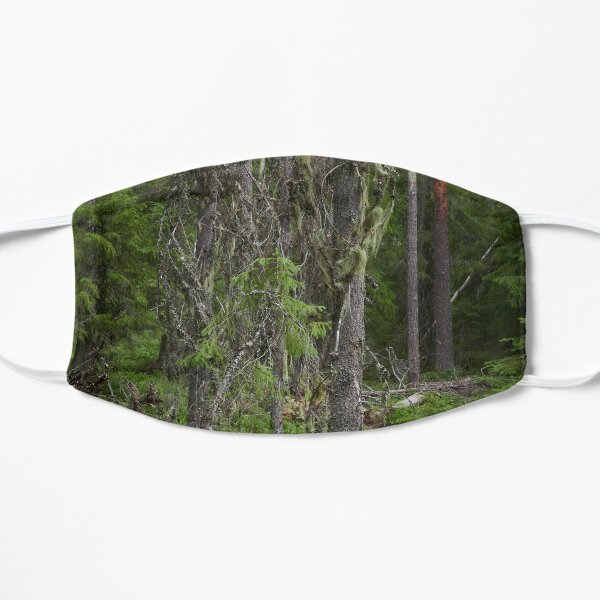The image is a vertically oriented photograph, showcasing a cloth mask commonly worn during the COVID-19 pandemic. The mask features an intricate and creative forest scene. Dead trees with barren branches and moss drape the foreground, while healthy pine trees with green needles are situated in the background. Additionally, the forest floor exhibits fallen logs and potentially ferns or low bushes, adding to the layered complexity of the scene. The mask's straps extend from each corner, and a small fold is visible on the right side. The mask stands out vividly against the plain white background, making the detailed forest imagery especially prominent.